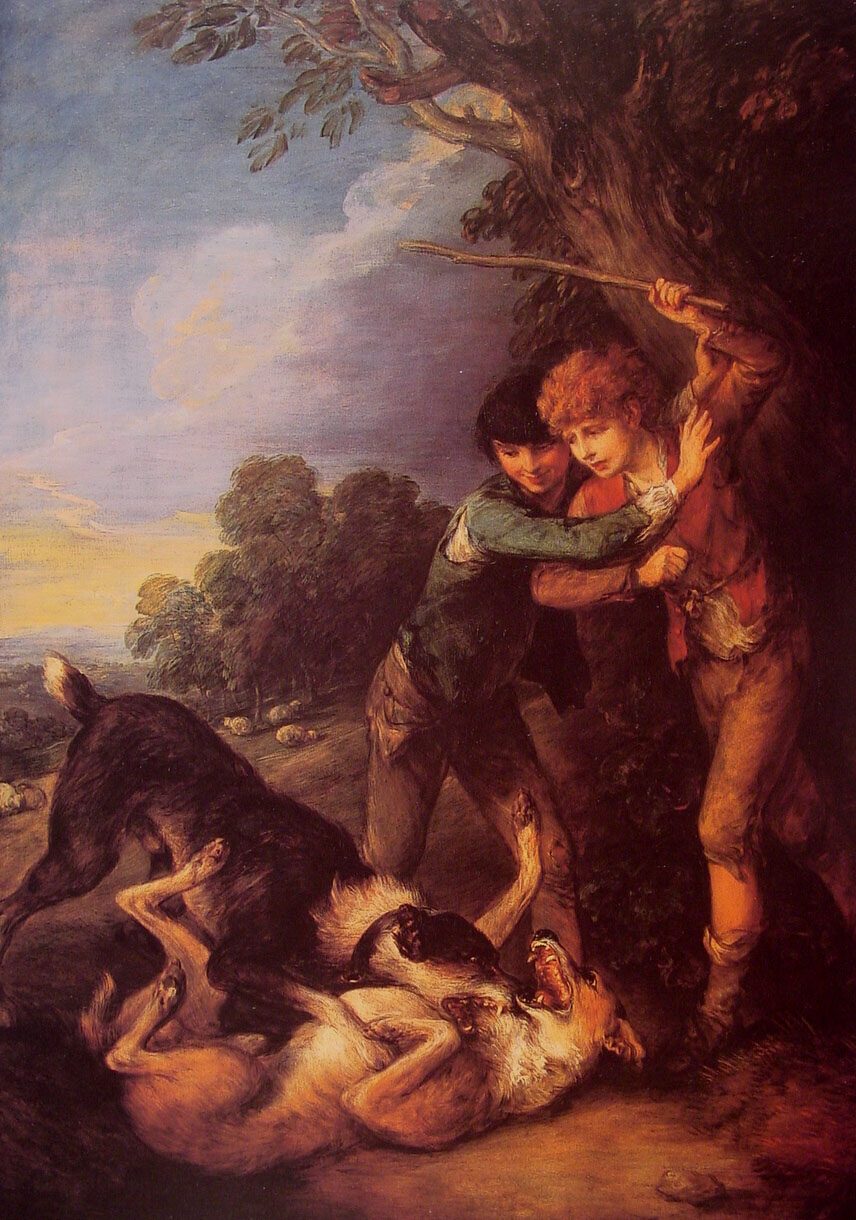This detailed painting portrays a dramatic scene featuring two shepherd boys and two dogs engaged in a fierce struggle. Positioned to the right side of the artwork, the boys stand under the shadow of a large tree, their expressions captured in a moment of intense emotion. The boy in the foreground, who has short curly red hair, is dressed in a red coat, white shirt, and tan pants. He holds a stick aloft, his face marked by worry as if ready to intervene and protect the dog he cares for. Next to him, attempting to restrain his friend, is a boy with short black hair and wearing a green shirt paired with light brown pants. His posture and grip suggest he believes the dogs might just be playing and wants to prevent any rash actions. 

At the boys' feet, two dogs are entangled in a confrontation. The tan and white dog lies on its back, mouth open in distress while the black and white dog aggressively pins it down, baring its teeth and aiming a bite towards the other dog’s throat. The black and white dog notably has a short tail. The rural setting is enriched with the background of a serene landscape featuring clear skies and additional greenery, but the focus remains firmly on the chaotic scene involving the boys and their dogs.